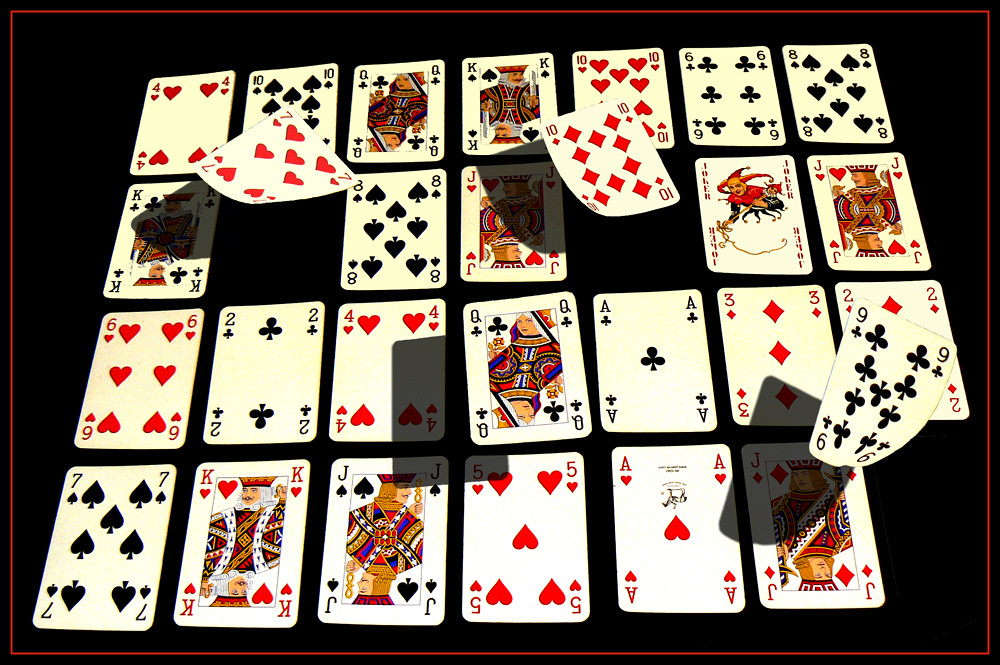This color illustration features a meticulously arranged display of playing cards, organized into four rows of seven cards each, set against a stark black background. Notably, four cards appear to be floating above the others, their edges slightly curved and casting shadows on the cards below, which emphasizes their elevation.

In the top row, the sequence of cards from left to right is as follows: the four of hearts, ten of spades, queen of clubs, king of spades, ten of hearts, six of clubs, and eight of spades.

The second row, also from left to right, contains: the king of clubs, a floating seven of hearts, eight of spades, jack of hearts, a floating ten of diamonds, joker, and another jack of hearts.

Moving to the third row, we see: the six of hearts, two of clubs, four of hearts, a floating eight of clubs, ace of clubs, three of diamonds, and two of diamonds.

Finally, in the bottom row, the cards from left to right are: the seven of spades, king of hearts, jack of spades, five of hearts, ace of hearts, jack of diamonds, and a floating nine of clubs.

Each card is evenly spaced within its row, enhancing the orderly and precise visual composition of the scene.